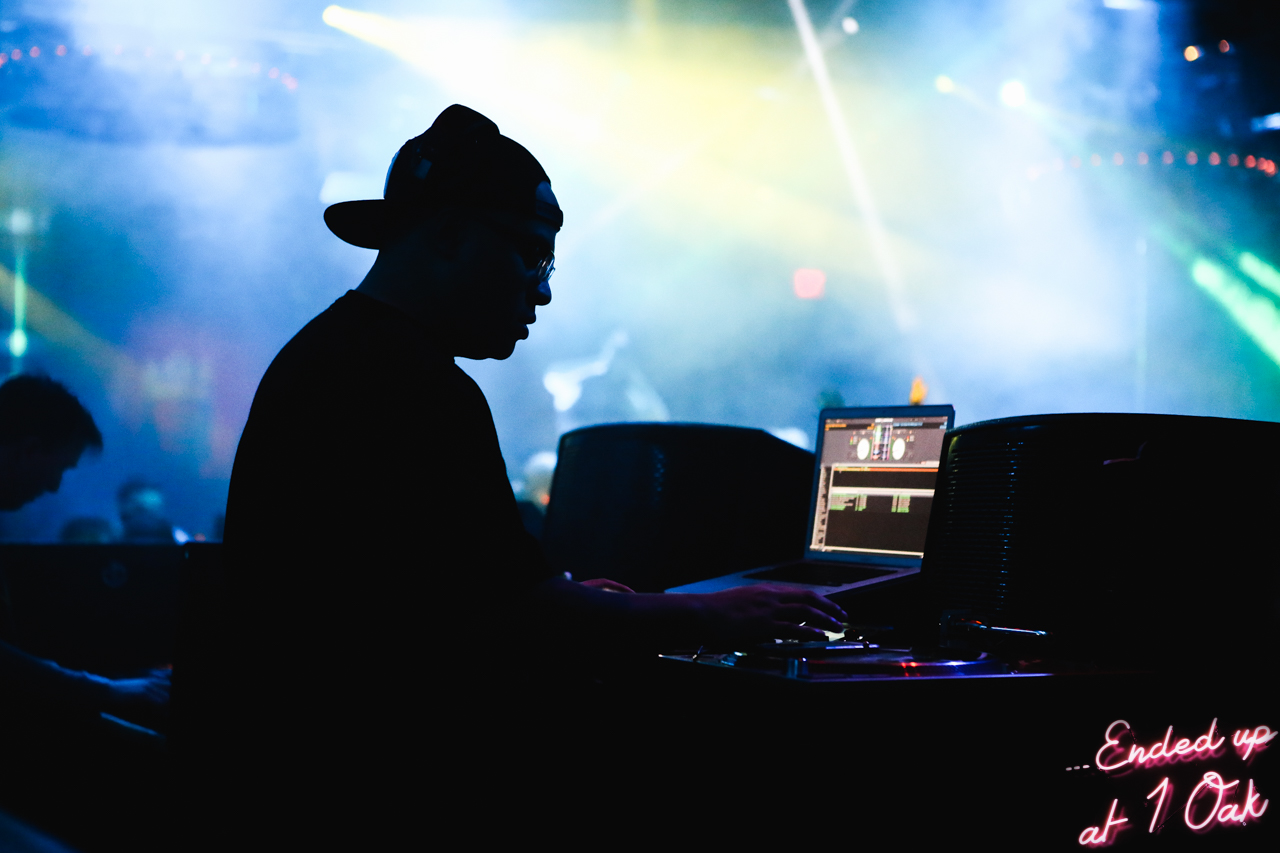In the dimly lit interior of a bustling dance club named "One Oak," a DJ stands in front of a glowing laptop, engrossed in his craft. The DJ, sporting a backward cap and sunglasses, is partially silhouetted by the vibrant strobe lights cutting through a hazy atmosphere filled with smoke. His right hand hovers over a turntable, suggesting he's manipulating digital records, while his other hand works on the laptop, which displays a music program filled with synthesizing commands and visualizations of spinning records. The backdrop features indistinct silhouettes of dancing patrons immersed in the pulsating energy of the club. In the bottom right corner of the image, red and white cursive text reads "...ended up at One Oak," subtly marking the location of this electrifying scene.